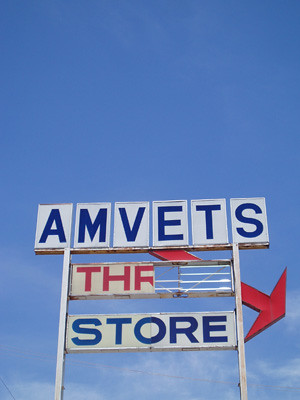This photograph captures a stark, clear sky with predominantly blue tones and a few wispy white clouds limning the lower half. Dominating the image is a weathered store sign that seems to have stood the test of time. The sign reads "AMVETS" in bold blue letters, each perched on its own sturdy white tile. Below, the word "THRIFT" once proudly displayed in red against white, is now truncated to "THR" as the remaining tiles have been lost with time. Further down, the word "STORE" appears in blue letters on a white background, with an arrow originating from the bottom of "AMVETS" and pointing diagonally towards the lower right. The structure is supported by two large posts that extend upward, curving past both sides of the sign. These posts intersect at the right end of the "A" in "AMVETS" and the left end of the "S," creating a unified frame.